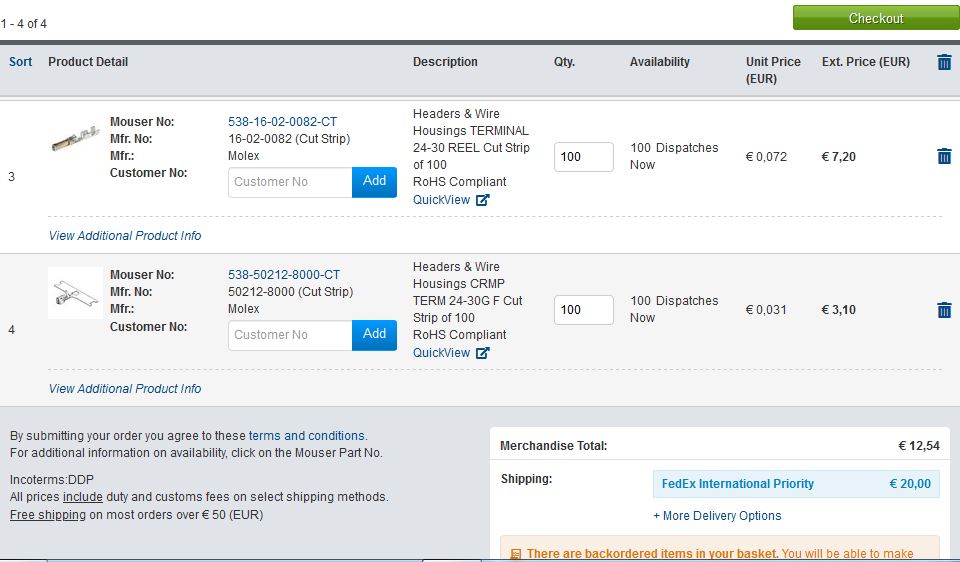**Image Description:**

The interface displays a section for checking out items from an online inventory.

- **Top Left Corner:**
  - Background is white.
  - Black text reads "1-404."

- **Top Center:**
  - A green rectangle with white text that says "Check Out."

- **Below the Check Out Button:**
  - A gray horizontal line extends across the section.
  - Below the line:
    - "Sort" is indicated in blue.
    - "Product Detail," "Description," "QTY," "Availability," "Unit Price," and "Total Price" are in black text.
    - A blue trash can icon appears.

- **Product Details Section:**
  - Quantity: "3"
  - Supplier: "Mouser" (abbreviated as "M-O-U-S-E-R")
  - Manufacturer Number: Abbreviated as "M-F-R" (Manufacturer) followed by several periods.
  - Customer Number: Abbreviated as "Customer No" followed by several periods.
  - Product Code: In blue text "5538-16-02-0082-CT"
  - Manufacturer Part Number: In black text "16-02-0282"
  - Item Description: "Cut Strip Molex"
  - Additional details: "Customer Number" notation is visible.
  - A blue background button with white text "Add."

- **Item Description:**
  - "Headlines and Wires, House and Terminal, 24 to 30 Rail"
  - "Cut Strip of 100"
  - Quantity labeled as "100 Patches"
  - Pricing details: "0.072" and "7.20"

- **Additional Icons and Links:**
  - A blue text link: "Additional Product Information".
  - A blue trash can icon.

- **Bottom Section:**
  - "Mergers Total: 1254"
  - Shipping Method: "FedEx International Priority"
  - Note: "More delivery options available."
  - Warning: "There are backorder items in your basket."

The image provides a comprehensive overview of the various product details and options available for managing items in the online shopping basket, emphasizing sort options, product information, quantity, and pricing details along with the necessary checkout actions.